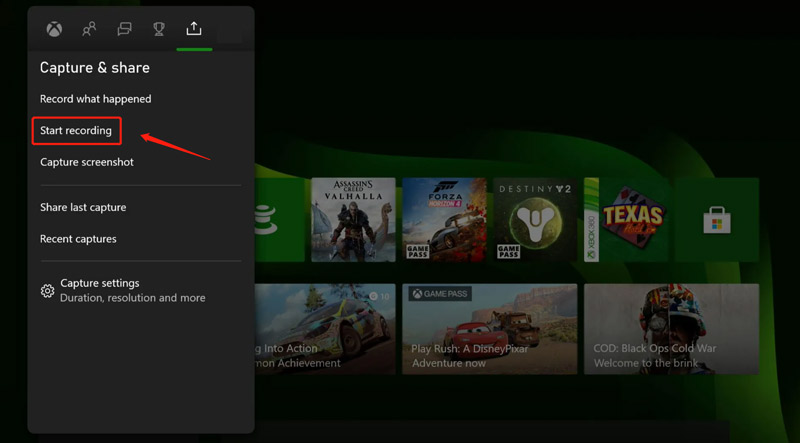This image features a software interface set against a black background. In the upper right corner, several icons are visible, including one depicting two people, another resembling a trophy, and an upward-pointing arrow. Below these icons, the text "Capture and Share" is displayed, followed by a prompt to "Record what happened." A red box with the text "Start Recording" is highlighted by a red arrow pointing towards it. Underneath, the options "Capture Screenshot" and "Share Last Capture" are listed, followed by "Recent Captures." Further down, a gear icon is accompanied by the text "Capture Settings," which includes options for "Duration," "Resolution," and more.

To the right of these settings are various video game covers. The first cover, for "Assassin's Creed Valhalla," features a man in armor wielding weapons in the foreground, with a ship equipped with a sail in the background. Moving right, the next cover is for "Forza," displaying a car amidst what may be fire, with "Game Pass" noted at the bottom of the cover. To the right of this is the cover for "Destiny 2," which showcases a large circle at its center and also includes "Game Pass" at the bottom. Next is a game with a green background adorned with playing cards, titled "Texas Hold'em."

On the far right, a green square displays the Microsoft logo. Below this section, additional game-related information is presented, including titles and phrases like "Game Pass," "Play Rush: A Disney Pixar Adventure Now," and "COD: Black Ops Cold War – Welcome to the brink.”